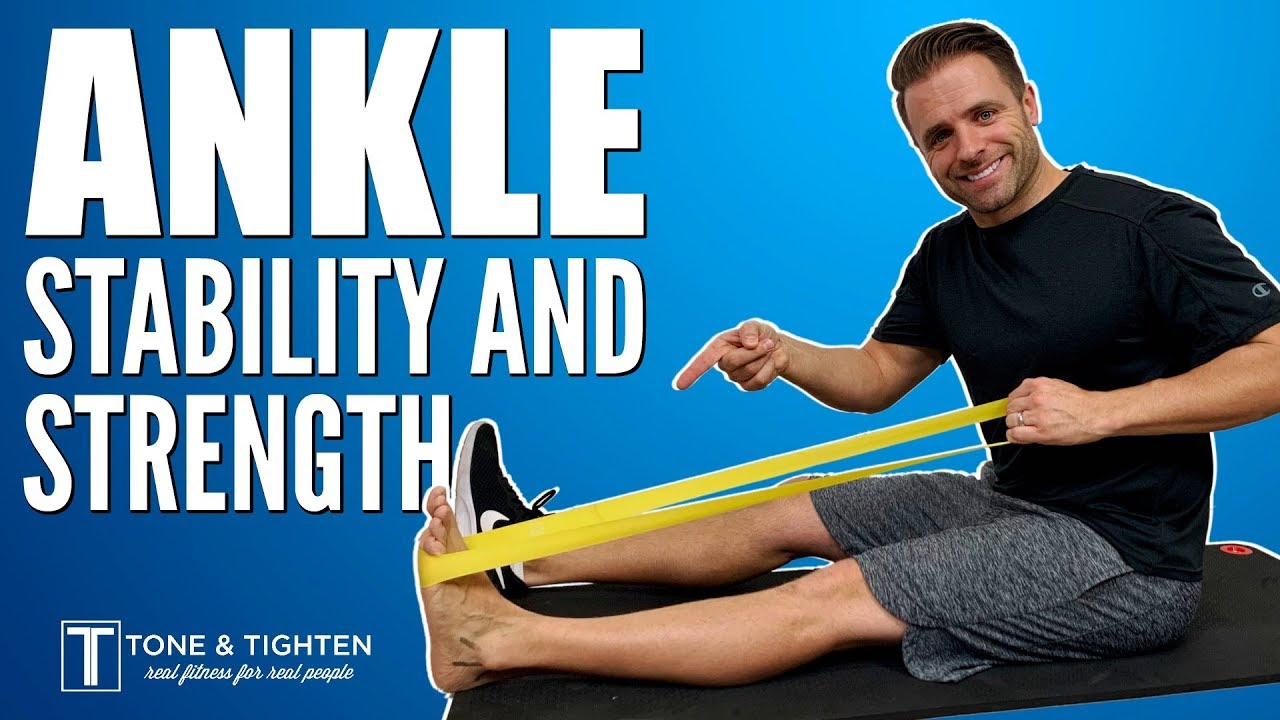The image is an advertisement for a product, featuring a gradient blue background that transitions from light blue in the top right corner to darker blue in the bottom left. Prominently displayed in bold, white text in the top left corner are the words "Ankle Stability and Strength." The bottom left corner contains the logo and slogan of the featured company, reading "Tone and Titan, Real Fitness for Real People," accompanied by a white letter "T" in a square.

On the right-hand side of the image is a photograph of a younger to middle-aged white man with brown, slicked-back hair, sitting on a black rectangular mat. He is dressed in a black short sleeve shirt and gray workout shorts. His right foot is adorned with a black Nike shoe featuring a white check mark and white soles, while his left foot is bare. Wrapped around his left foot is a yellow flexible workout band, which he is holding and stretching about two and a half to three feet with his left hand. He is pointing at his left foot and smiling, emphasizing the focus on ankle stability and strength. A thin white border frames the photograph to make it stand out against the blue background.